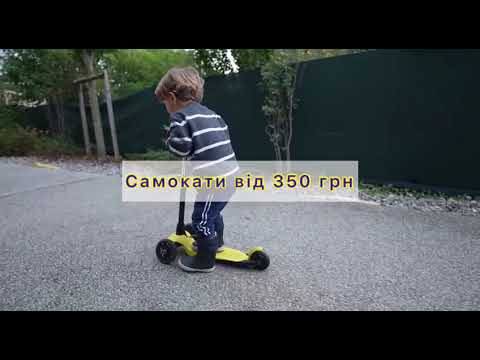In this vibrant and detailed photograph, a young boy, approximately four years old, is captured in the middle of riding a yellow tricycle-style scooter with two front wheels and one back wheel. The boy, who has brown hair, is wearing navy blue sweatpants with white stripes down the sides, a dark grey long-sleeved shirt adorned with white horizontal stripes, and black rubber boots. His scooter features a black handle. He rides along a greyish street sidewalk, with a green mesh fence and trees forming the natural backdrop to his right. A wooden post and trimmed green hedges add to the scenery, under a sky that appears grey. At the top of the photograph, a white rectangle with black and yellow text, which seems to be in Russian or another foreign language, includes the letters "C-A-M-O-K" followed by additional characters and numbers "350-R-P-H." The vibrant colors and detailed elements of the scene, combined with the foreign text, give the image a vivid and dynamic atmosphere.